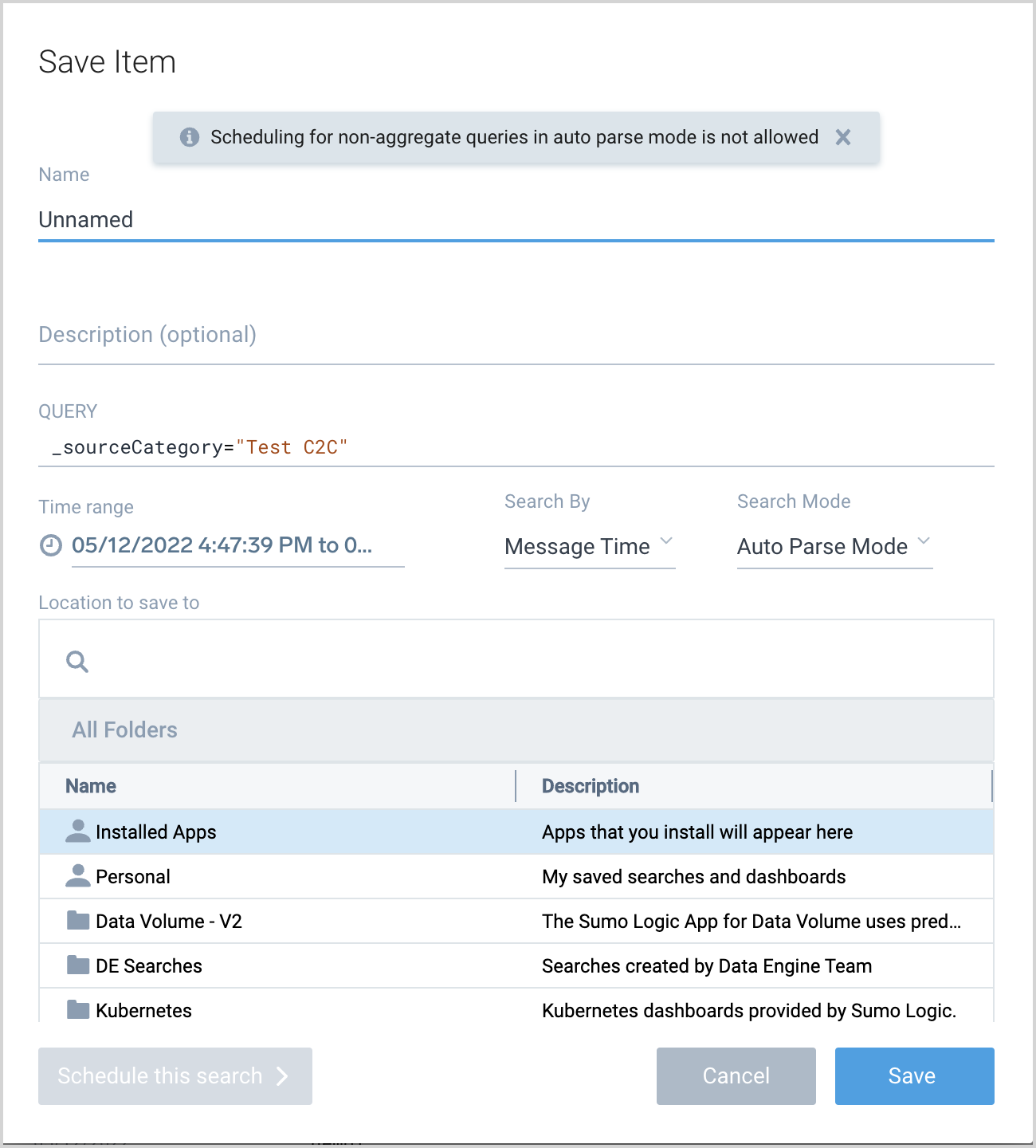This image is a cropped screenshot from a web page, showing a setup window for saving queries. The top line displays the option "Save Item." An alert is prominently featured, stating, "Scheduling for non-aggregate queries in AutoPass Safe Mode is not allowed." The item being saved currently has no specified name and is labelled "Unnamed." The window contains a written query, a specified time range, and an option to select a saving location for the query. The available folders for saving include "Installed Apps," "Personal," "Data Volume V2," "DE Searches," and "Kubernetes." The setup appears to be designed for managing and automatically running queries.